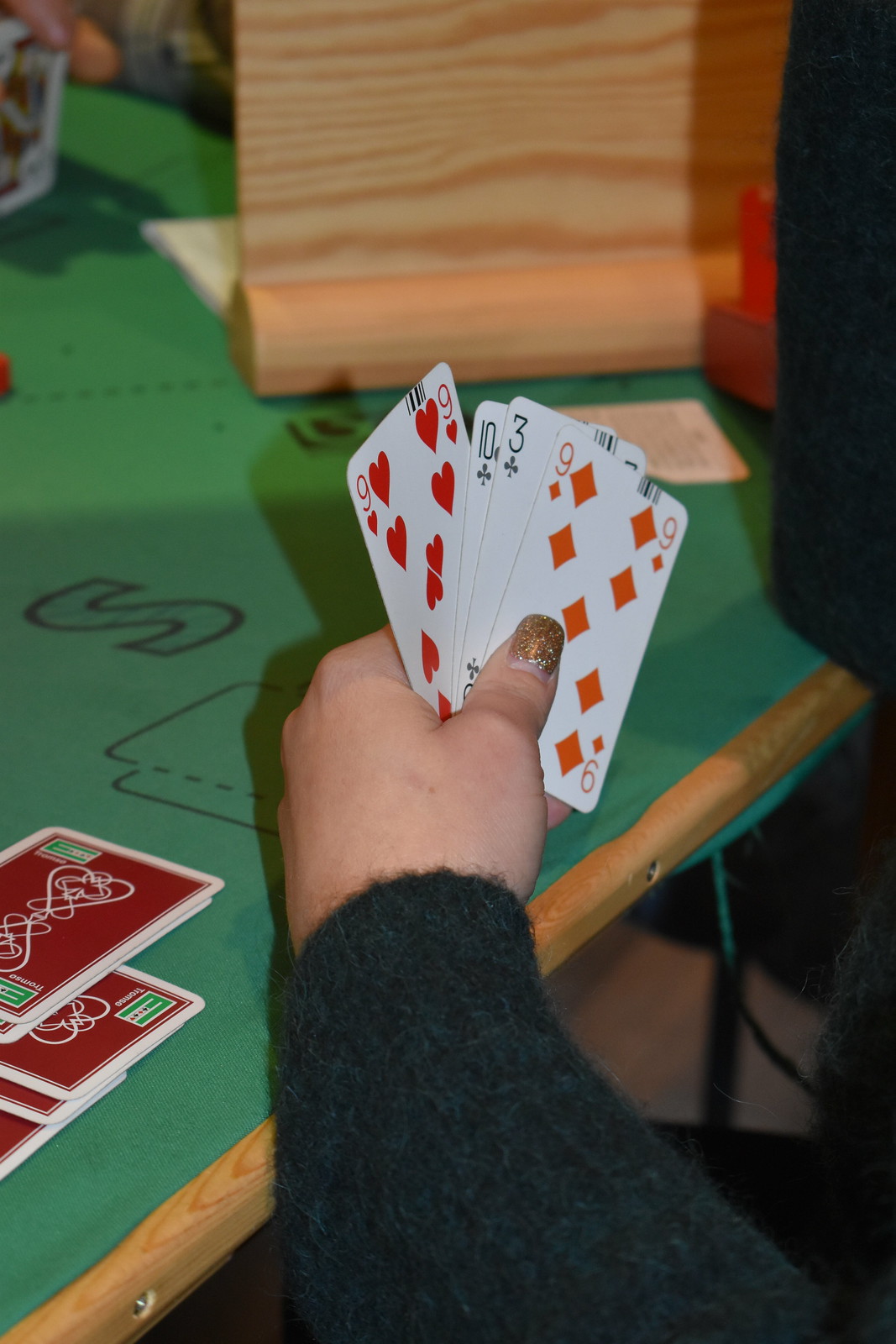A man is seated at a casino table, which is covered with green felt. Prominently, the table features a large, stylized letter "S" and an illustration of cards delineated by broken lines beneath it. A hand, appearing female due to its colored thumb, is positioned on the table, holding a fan of cards: the Nine of Hearts, Ten of Clubs, Three of Clubs, and Nine of Diamonds. In the bottom left corner, five cards lie face down, their faces obscured. The person is dressed in a black, long-sleeved knitted shirt. Above this hand is a wooden divider, likely meant to obscure the player's hand from other competitors. In the top left of the image, another hand is visible, holding what seems to be the Jack of Clubs.